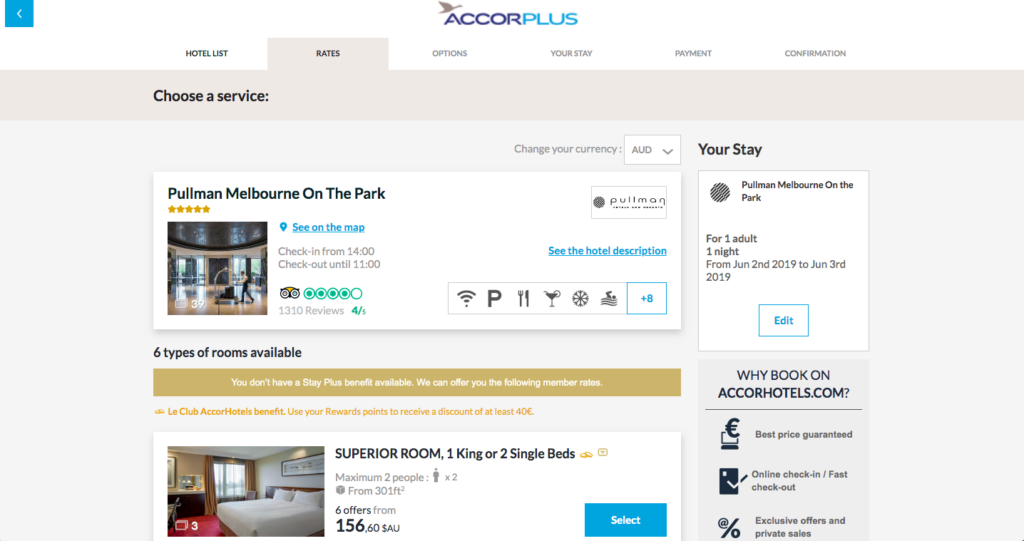The image is a detailed traveling booking interface for Pullman Melbourne on the Park, observed on a booking site (possibly AccorHotels.com).

In the top left corner, there’s a blue banner with an "Accor Plus" logo. Adjacent, another section returns you to the hotel listings. Below, a gray tab displays options such as rates, USG, payment, and confirmation. A large gray rectangle features commands to choose a service or change your currency.

Highlighted is Pullman Melbourne on the Park, represented by five gold stars, and a specific prompt, "C on the map.” The check-in time is from 14:00, while check-out is until 11:00. The TripAdvisor logo shows four green circles based on 30 to 10 reviews.

Further details reveal the booking specifics for Pullman Melbourne on the Park: 
- For one adult, one night
- Dates from June 7, 2019, to June 3, 2019
- The booking guarantees the best price, online check-in, and private check-out on AccorHotels.com.

The hotel benefits include good options for walkers and private accommodations. Six room types are available, highlighted with gold rectangles and white text, prominently featuring superior rooms with various configurations (one king bed or two single beds) for up to two people. Additional description includes red carpets, white beds, brown and white walls.

AccorHotels benefits include earning user rewards points to receive a discount of at least 40 euros. Members can access special rates and additional perks. Room images showcase comfortable amenities, indicated as "Superior Room, with one king or two single beds." The caption also mentions offers ranging between six cents to six stars a year, though this part is slightly ambiguous.

Overall, the image concisely shows the luxurious nature of Pullman Melbourne on the Park and the enhanced booking benefits offered through AccorHotels.